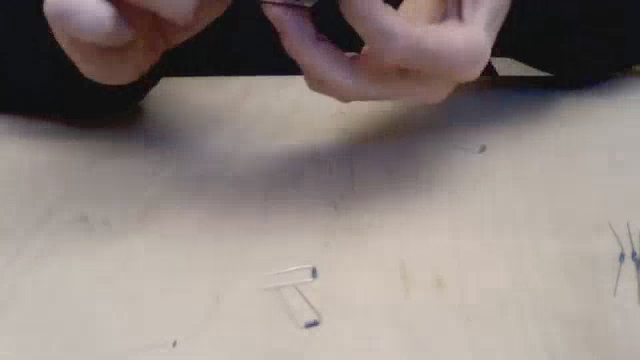The grainy, horizontally cropped snapshot captures a pair of Caucasian male hands, identifiable by their black long-sleeved attire. The hands dominate the top section of the image, with the left hand's fingers curled inward and the right hand curled under. The man is seemingly engaged in delicate work as his forearms rest on a white surface, which could be a tablecloth or a tabletop. Below his hands are several partially visible objects: two transparent rectangles with black squiggles at the ends and two identical small cylindrical components, possibly resistors, each with two wires extending from either end. Additionally, two bent-wire resistors form a U-shape, positioned just below the hands. The overall scene suggests the man is manipulating electronic components, though the image's low contrast and blurry quality obscure the finer details.